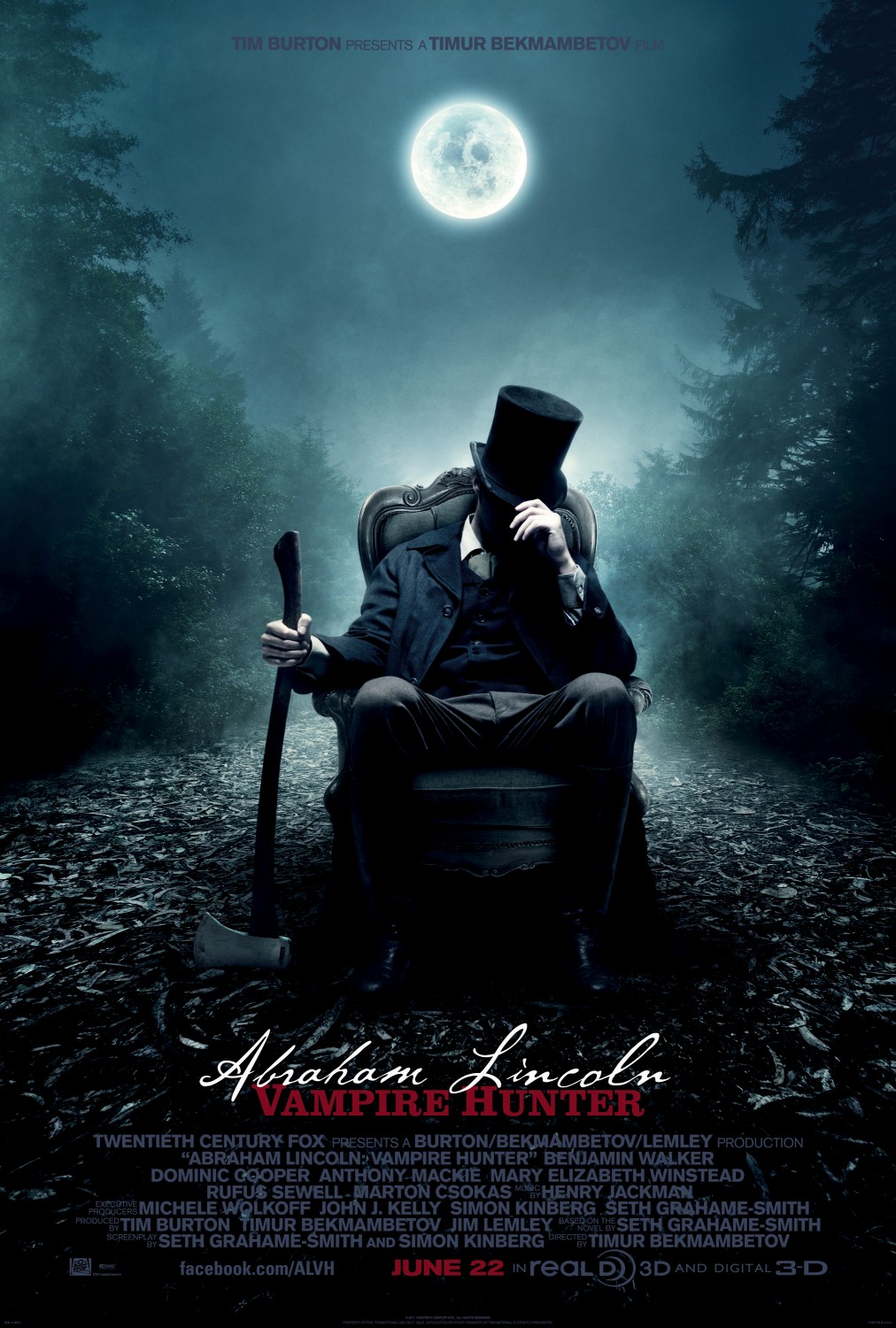The movie poster for "Abraham Lincoln: Vampire Hunter" is set against a chilling night-time backdrop characterized by an eerie dark forest. The scene is illuminated solely by the glow of a full moon, casting a ghostly light over the surroundings. Abraham Lincoln, dressed in a black suit and wearing his iconic top hat, occupies an old-fashioned armchair positioned on a path that stretches into the dark forest. With his head bowed and the brim of his hat pulled down to obscure his face, Lincoln presents a brooding and mysterious figure. In his right hand, he holds the haft of an axe, its head resting on the ground. The forest floor is strewn with dead leaves, enhancing the sinister ambiance. The poster's text features "Abraham Lincoln" in a white cursive script, with "Vampire Hunter" in a Gothic serif font below. Additional text in dark gray provides production details and credits, while the release date, June 22nd, stands out in red. Logos for Reel 3D and Facebook are also included at the bottom, indicating the movie's 3D release and social media presence. This atmospheric poster from 20th Century Fox effectively sets the stage for the macabre adventures of Lincoln as a vampire hunter.